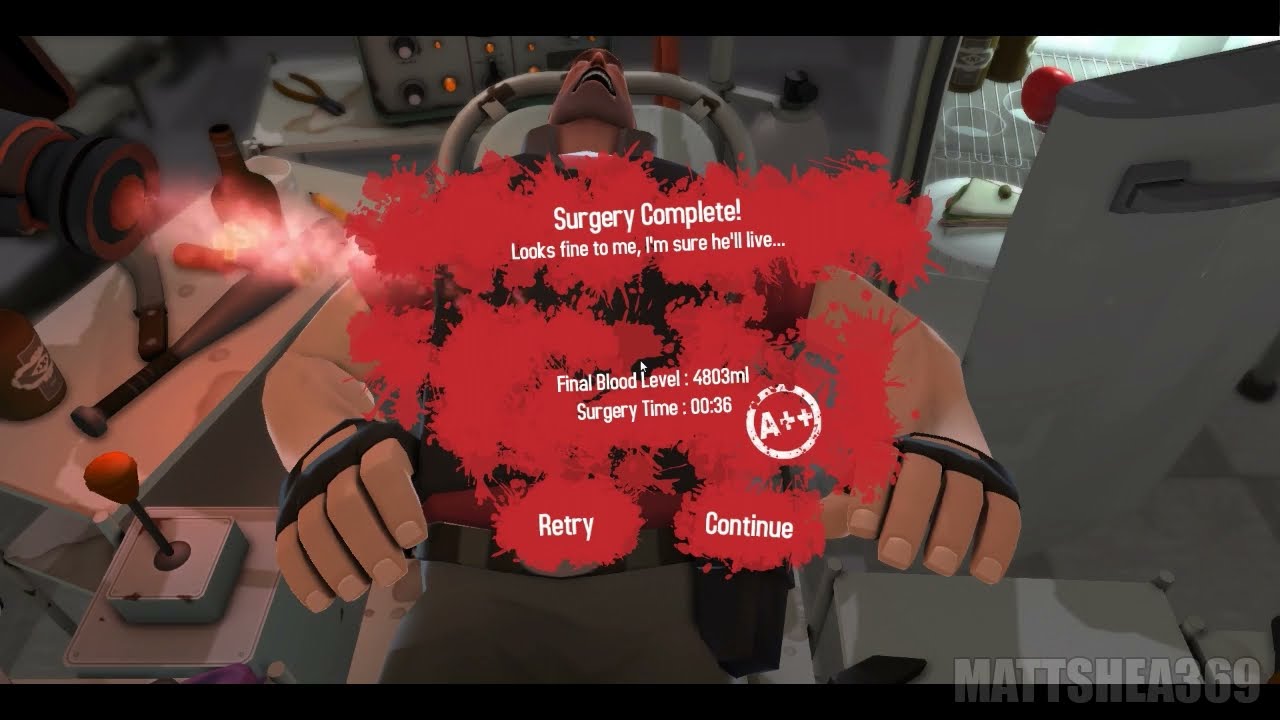The image is a detailed screen capture from a 2D animated video game, centered around a character lying on a gurney with his face upward and eyes closed. The man is large, with very large arms, and his skin is light brown. He is wearing tan pants, a belt, and fingerless gloves. Above him, the screen displays red, bloody text that reads in white letters: "Surgery complete. Looks fine to me. I’m sure he’ll live..." Below this, additional text reports: "Final blood level, 4803 milliliters. Surgery time, 36 seconds. A++."

The environment around the gurney is filled with an assortment of objects. On the left-hand side of the screen is a white table holding unconventional medical tools such as knives, alcohol bottles, what appears to be a machete, and a baseball bat. Behind the man, a radio with flashing buttons is visible. To the right, an open refrigerator with no food in it can be seen, the door slightly ajar. Also in the lower part of the screen, there are options for the player to "retry" or "continue."

Additionally, in the lower-right corner of the screen, there is a watermark: "MatsHe369", indicating the creator of the screenshot. The color palette consists of gray, light brown, white, and red. There are no other characters or animals present in the image.